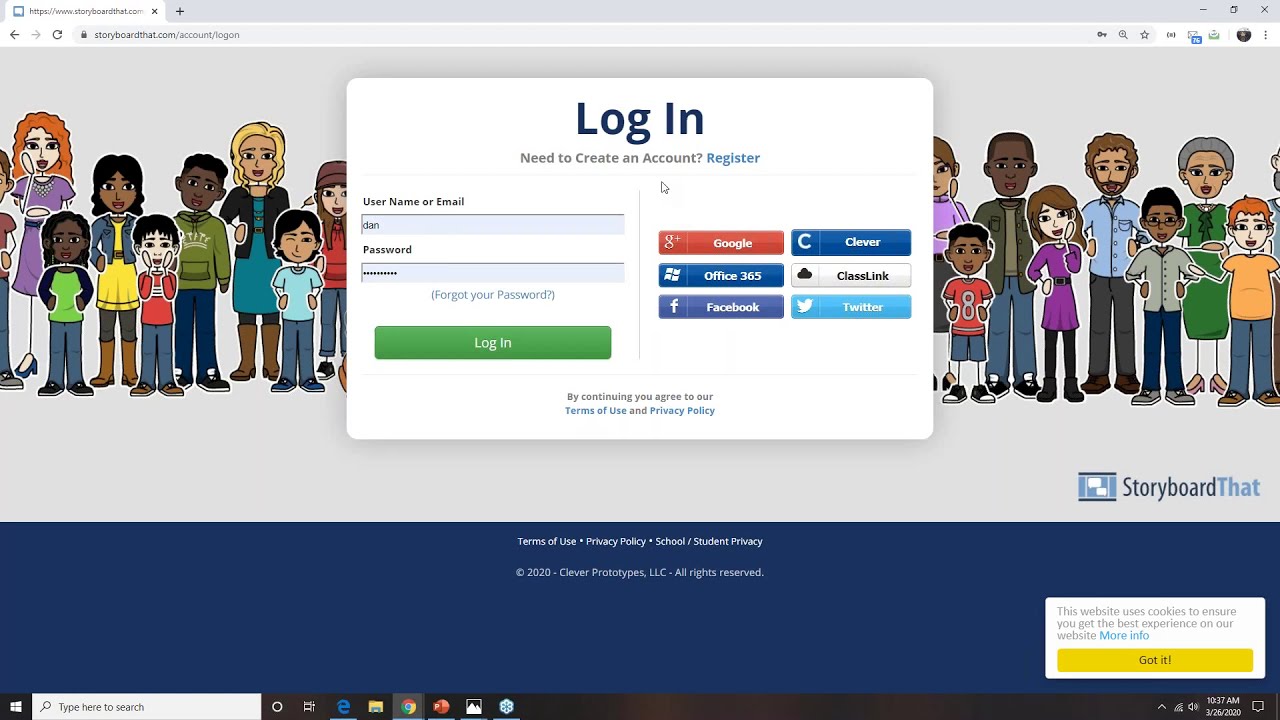The image depicts the login page of the website "Storyboard That," accessible via the URL https://www.storyboardthat.com/account/logon. The URL is clearly visible both in the address bar and on the webpage tab. The background features an array of cartoon characters, representing men, women, and children of various ages, sizes, and dressed in colorful attire.

In the center of the screen, there is a white rectangular pop-up box, oriented horizontally, prompting the user to log in. At the top of the pop-up, the text "Log In" is prominently displayed, followed by a smaller-font prompt that reads, "Need to create an account? Register," in blue. Below this prompt is a form field labeled "Username or E-mail," pre-filled with the text "Dan." The subsequent field is labeled "Password," although the password input is obscured for security purposes. Beneath the password field is a "Forgot your password?" link in gray.

A large green "Log In" button is positioned beneath this form. To the right of the pop-up, there are icons for alternative login options, including Google, Office 365, Facebook, Clever, ClassLink, and Twitter. At the very bottom of the pop-up is a disclaimer that reads, "By continuing, you agree to our terms of use and privacy policy."